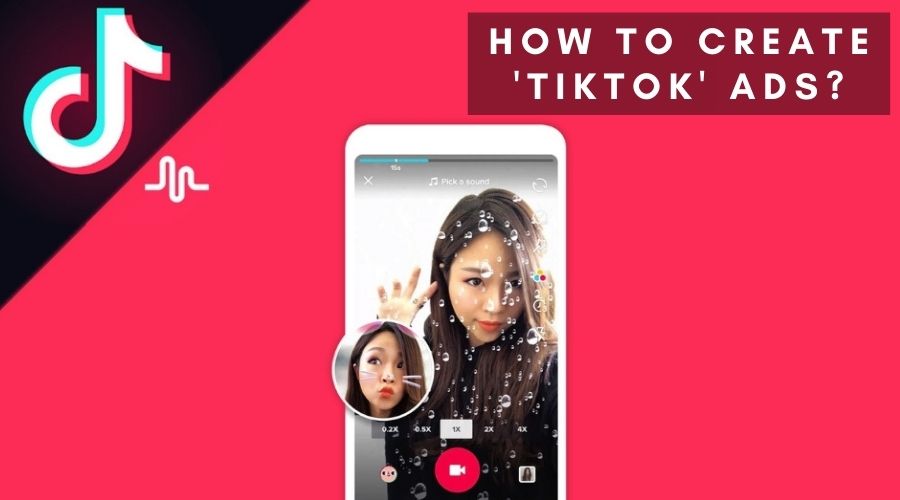The image is designed for TikTok and features a dominant pink rectangle as the background. In the top left corner, there's a black triangle containing a logo composed of blue, white, and pink colors. Adjacent to this black triangle, within the pink area, is another small logo resembling a bent pipe.

At the center of the image, a smartphone displays an Asian girl who appears to be looking down at the screen. The smartphone also shows a smaller, circular image of the same girl with a cat's face filter applied.

In the top right corner, a red rectangular banner features bold white capital letters that read, "HOW TO CREATE 'TIKTOK ADS'." The overall composition includes the prominent pink background, a black triangle with a logo in the top left, a red rectangular banner with text in the top right, and a centrally placed smartphone with images of the girl.